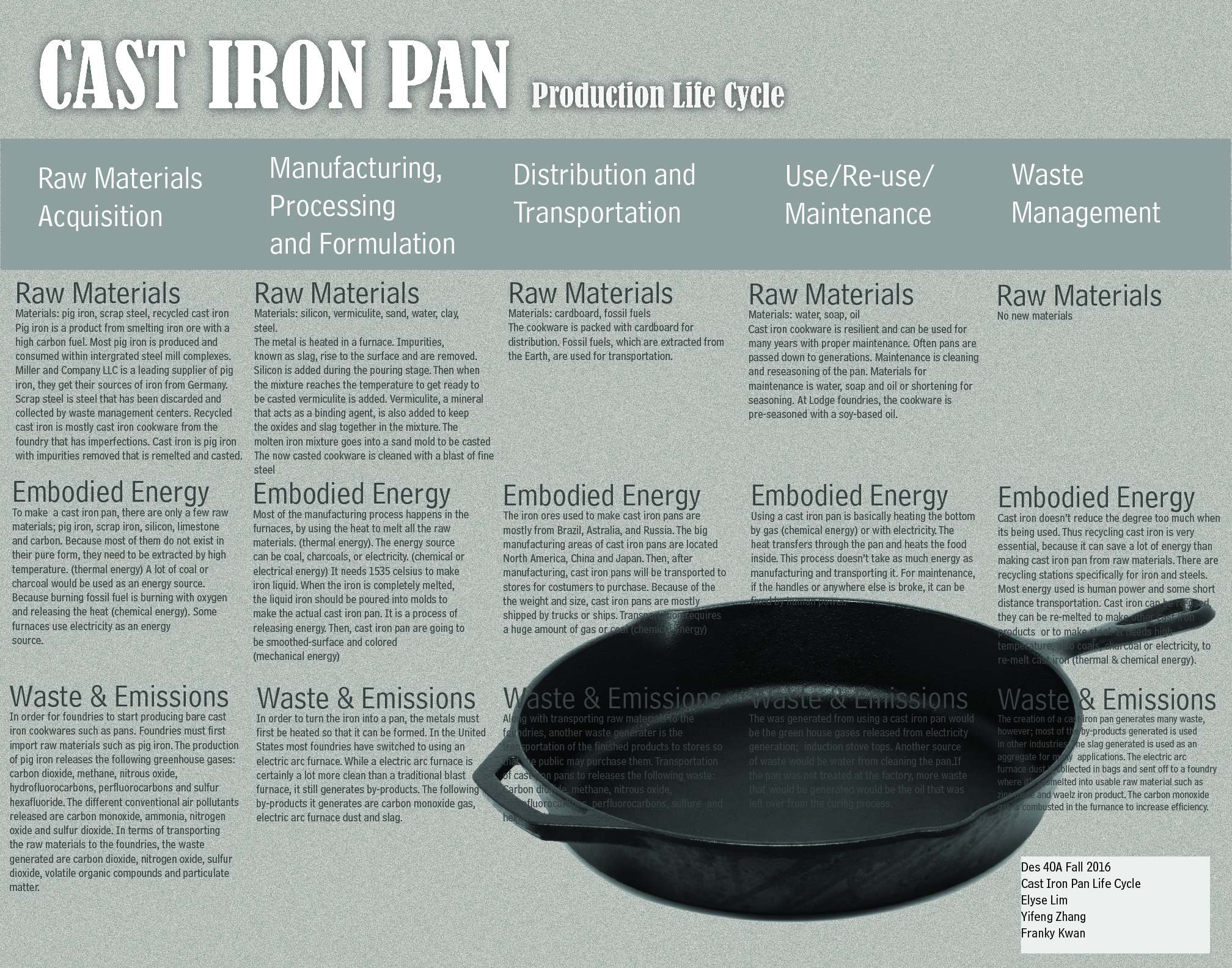The image features an informational sheet with a gray background, displaying detailed content about the production life cycle of a cast iron pan. At the top, large uppercase bold letters spell out "CAST IRON PAN," and directly beneath in smaller letters, "Production Life Cycle" is written. Below, the sheet is divided into five columns, each topped with white font headings reading: Raw Materials Acquisition, Manufacturing, Processing and Formulation, Distribution and Transportation, Use, Reuse, Maintenance, and Waste Management. Each of these columns contains several informational paragraphs, each with its own bold, large-font subheadings labeled: Raw Materials, Embodied Energy, and Waste and Emissions. In the lower right-hand corner, the sheet features an image of an empty cast iron skillet, providing a visual reference to the subject matter. The document serves as a comprehensive overview of the various stages involved in the lifecycle of a cast iron pan.